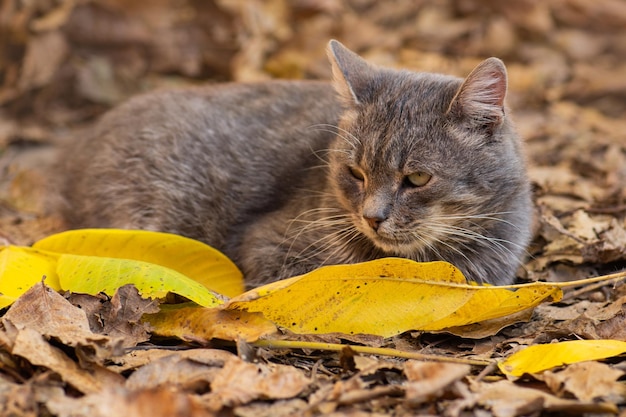This photograph captures a striking gray and white cat amidst a bed of dry fall leaves, with the background fading into a soft blur. The cat, which takes up most of the image, is curled slightly with a watchful yet sleepy gaze, peering to the side with partially closed, greenish-yellow eyes. Its perked ears and long white whiskers add to its alert expression, despite the apparent drowsiness. The cat's fur appears short and clean, and its nose features a touch of pink. Surrounding the feline are primarily old, brown decomposing leaves, but prominently in the foreground stretch vibrant, large yellow leaves nearly spanning the width of the picture.